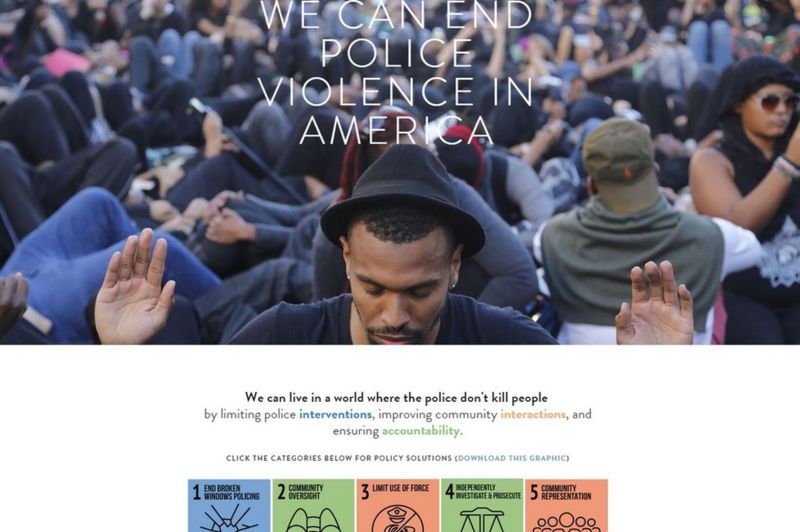Detailed Caption:

The image is a powerful political poster advocating for an end to police violence in America. It features a widescreen photo of a large crowd, focusing on an African American man at the forefront. The man, with short hair and wearing a sleek black fedora, stands with both hands raised in a gesture of surrender or solidarity. Adorned with earrings, his face is partly obscured as the image cuts off at his chin, and he appears to be looking downward in a poignant moment of reflection. 

Positioned above his hat, bold text declares, "We can end police violence in America." Below the image, further text outlines a hopeful vision: "We can live in a world where the police don't kill people by limiting police interventions, improving community interactions, and ensuring accountability." The call to action invites viewers to explore policy solutions, directing them with the prompt, "Click the categories below for policy solutions," followed by an invitation in blue hypertext to "download this graphic."

At the bottom, a series of five clickable graphic icons in shades of blue, mossy green, and melon orange presents specific reform measures. These measures include: 
1. End Broken Windows Policing.
2. Community Oversight.
3. Limit Use of Force.
4. Independently Investigate and Prosecute.
5. Community Representation.

Each icon is numbered and color-coded, providing a user-friendly guide to actionable steps aimed at curbing police violence.